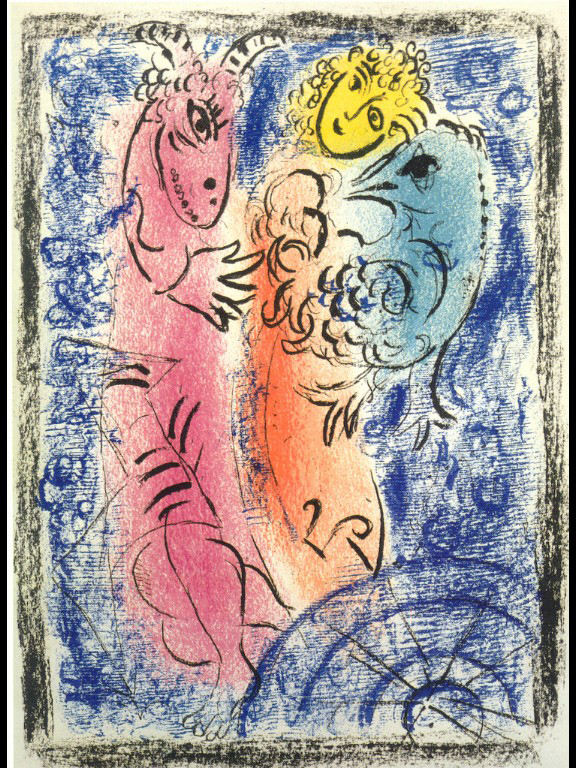This vibrant piece of art, seemingly from a coloring book and likely colored by a child, features a striking composition of fantastical creatures and abstract elements drawn and filled in with crayon or charcoal. Framed by a thick black border, the vertically aligned rectangular artwork organizes its elements with a central, yellow-faced woman's visage, outlined in black with curly hair and expressive features.

To the left of the woman's face is a red, perhaps pink, slender creature with humanoid qualities, notably a human-like hand and elongated eyelashes. This creature's facial features include white, dashed horns and a small, circular nose, rendering it both whimsical and otherworldly. Its red hue extends downward, merging with hints of darker shades.

To the right of the yellow face, a blue figure that could be a bird or a baby dinosaur displays a sharp beak and a pronounced eye, suggesting it's tenderly held by the central figure. The creature's blue extends into the circular, scribbly lines of blue that swirl throughout the background, providing a sense of movement and depth.

Overlaying these vibrant characters are swirling patterns that consist of circular dark blue lines, creating an almost hypnotic backdrop. The entirety of this scene is edged with the black crayon or charcoal lines, forming a border that ties the eclectic elements into a cohesive display of imaginative art.